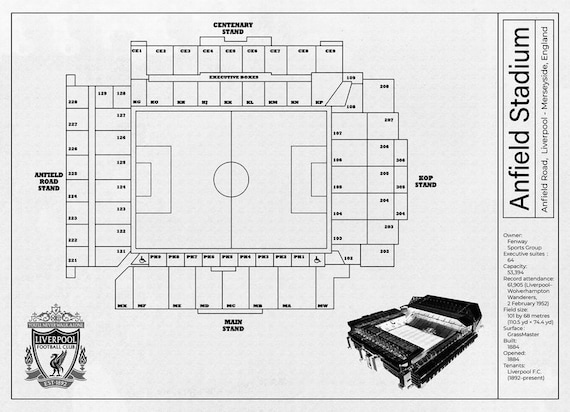This detailed diagram of Anfield Stadium, labeled vertically on the right side of the image, meticulously outlines the layout and key features of Liverpool Football Club's home ground, located at Anfield Road, Liverpool, Merseyside, England. The central section prominently displays the stadium's seating chart, featuring the Centenary Stand at the top, Anfield Road Stand on the left, Main Stand at the bottom, and KOP Stand on the right. Key details such as the Executive Suite capacity of 64 and the stadium’s total capacity of 59,894 are noted, along with other pertinent stadium statistics like field surface and opening date, though some specifics are obscured. Adjacent to the diagram, a black and white image depicts the stadium, capturing the bleachers and overall architecture. At the bottom left corner, the Liverpool Football Club logo is displayed on a crest, with the team's founding year, "EST 1892," clearly visible underneath.